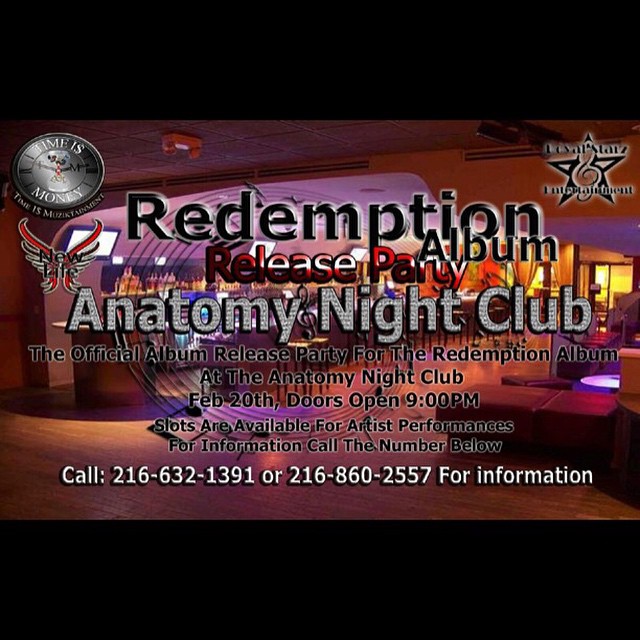The image is a promotional advertisement for the "Redemption" album release party at Anatomy Nightclub. It has solid black bars at the top and bottom framing an interior view of the nightclub, which features a vibrant, festive atmosphere with purple and yellow lighting. In the middle, the club's bar area is visible, showcasing numerous alcohol bottles, bar stools, and a hardwood floor, with a lounge area to the right. 

Text overlays the image, primarily with the event details. In bold black letters, it reads "Redemption Album," followed by "Release Party" in red and white. Below, it highlights "Anatomy Nightclub" in a graphic, diamond-like font. The event is described as the official album release party for the Redemption Album, scheduled for February 20th. Doors open at 9 p.m., and slots are available for artist performances. Contact information is provided with two phone numbers: 216-632-1391 and 216-860-2557.

Additional logos decorate the image: a silver "Time is Money" coin in the top left, a red "New Life" emblem with wings just below it, and in the upper right, a musical note with a star. The overall design typifies a nightclub promotional flyer, blending bright, flashy graphics with detailed event information.